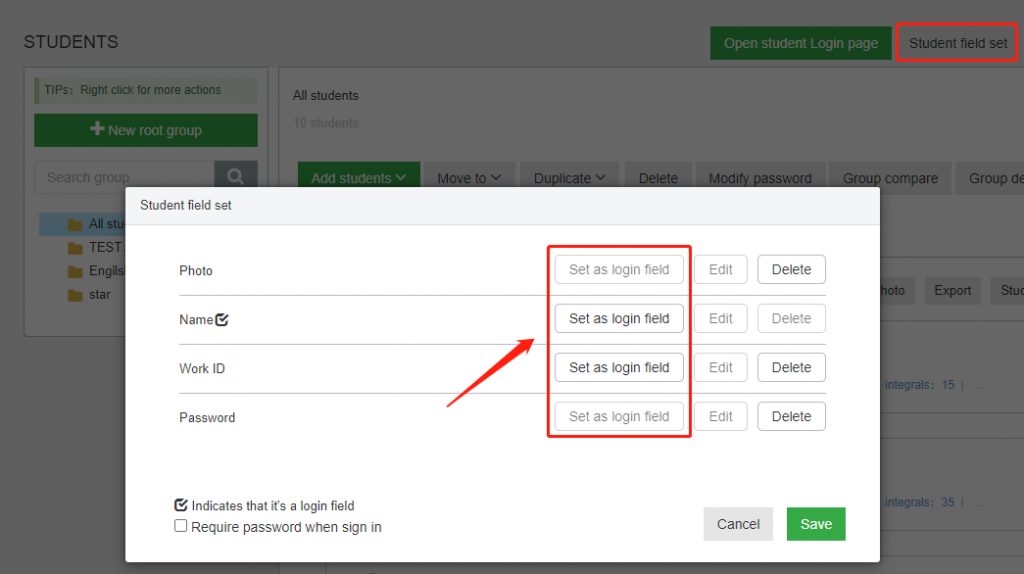The image depicts a student management interface designed for teachers. The background is grayed out, making the interactive elements stand out prominently. On the left side of the page, the word "Students" is displayed in large text. Below this title is a conspicuous green box labeled "New Root Group," alongside several obscured, unreadable folders.

The most eye-catching part of the interface is the "Student Field Set" section, a bright white area subdivided into four fields: Photo, Name, Work ID, and Password. Each field has three associated actions: "Set as Login Field," "Edit," and "Delete." The "Set as Login Field" option is highlighted with a red rectangle and accompanied by a red arrow, drawing immediate attention. At the bottom of this section, there are also "Cancel" and "Save" buttons, with the "Save" button colored green.

In the blurred background, multiple buttons are visible, each labeled with functions such as "Add Students," "Move To," "Duplicate," "Delete," "Modify Password," "Group Compare," and "Export." However, these options are currently inactive due to the focus being on the "Student Field Set" section.